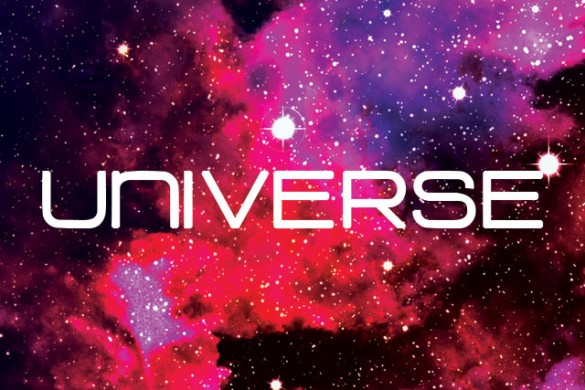This horizontally aligned rectangular image, approximately four inches wide and three inches tall, presents an otherworldly sky bursting with color. The center features the word "universe" in large, bold, white sans-serif font stretching from left to right. The sky itself transitions through a spectrum of hues: beginning with black scattered with tiny white specks in the upper left corner, morphing into shades of pink and purple toward the middle and upper right sections, and mixing again with black and pink in the lower right-hand side. White dots, representing stars, are dispersed throughout the backdrop, with sizes varying from minuscule to medium, and a few distinctly larger ones. Notably, two of the largest dots—embellished with flare bursts—are positioned just above the V and E, and the last E in "universe," seeming to emphasize the celestial theme of the image. The vibrant pink, purple, and black clouds amidst the stars evoke a sense of an abstract or imaginary outer space, filled with cosmic gases and stellar wonders, making it hard to discern whether it's a photograph or a digitally constructed image.